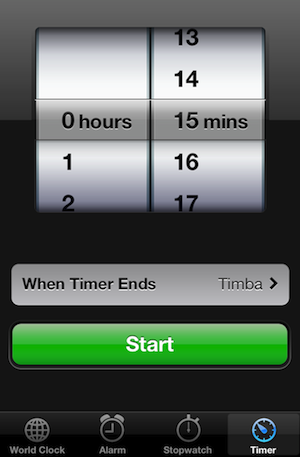This image showcases a simple, gray-colored timer interface. The layout is organized and minimalistic, with various time-related functionalities.

On the left side of the interface, there's a vertical list of numbers representing hours, starting from zero at the top, followed by one and two. Correspondingly, on the right side, a similar vertical list displays minutes starting from 13, then 14, 15, 16, and 17. 

Below these numbers, there is a text that reads "When Timer Ends." Adjacent to this text, an arrow points to the right, and the word "Timbre" is displayed, presumably indicating a sound option.

At the center of the interface, a prominent green bar with the word "Start" in white text invites users to begin the timer.

Functionality icons are lined up horizontally at the bottom of the interface. From left to right, they are:
- World Clock
- Alarm (depicted with an icon of a clock)
- Stopwatch
- Timer 

Each icon is clearly labeled to indicate its function, providing a user-friendly experience.